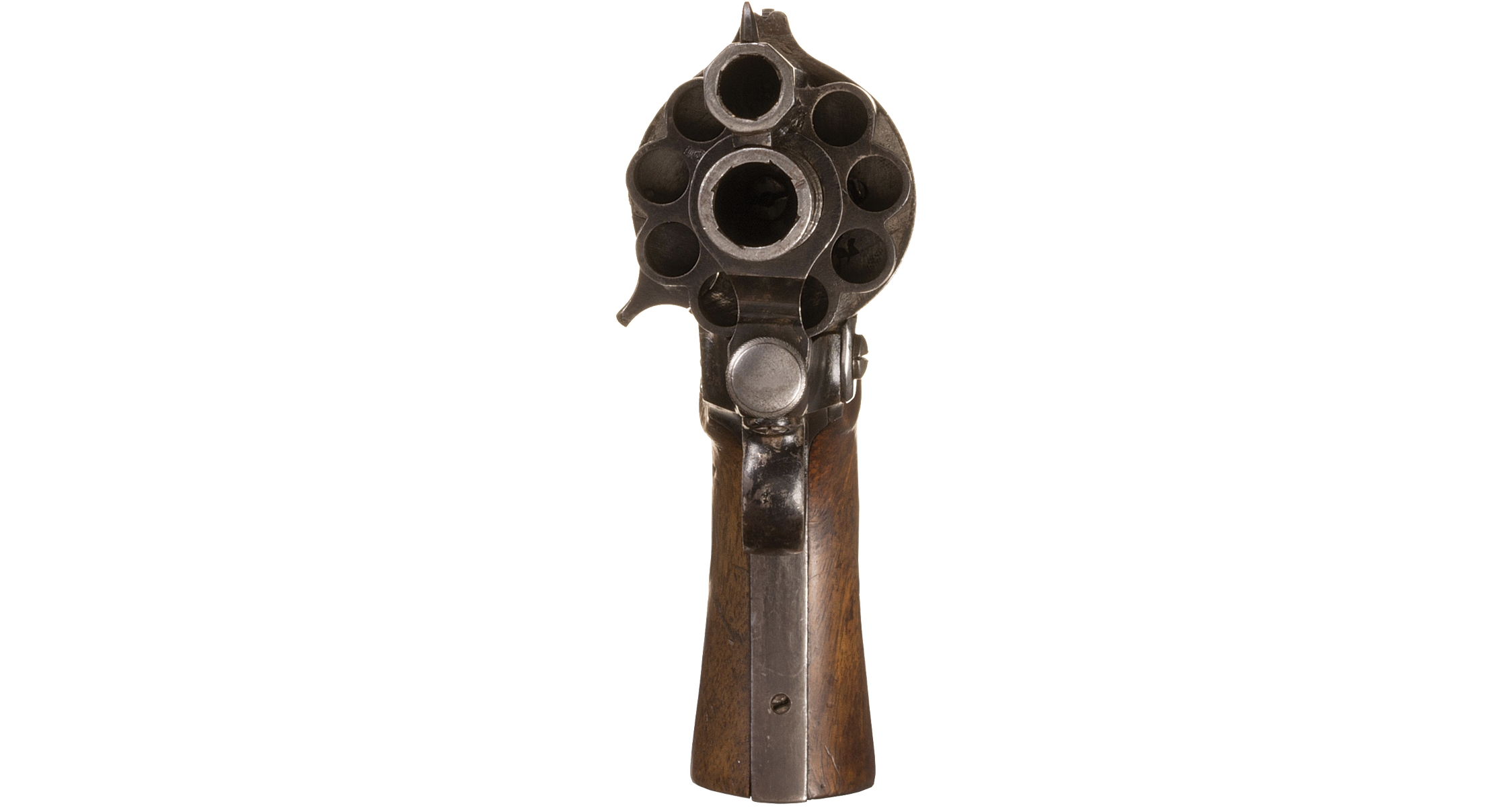This image showcases a close-up front view of a revolver against a completely white background. The revolver dominates the frame, with particular emphasis on its empty bullet chambers, highlighting the metallic, cylindrical area where rounds would be inserted. The metallic parts of the revolver are primarily grey, with some darker iron-like areas displaying six smaller circles and two larger circles, all without bullets. The detailed craftsmanship of the revolver is evident with its wooden and brown grip, contrasting the sleek, metallic components. Visible elements such as the muzzle, trigger guard, and various metal rings enhance the intricate design of this firearm.